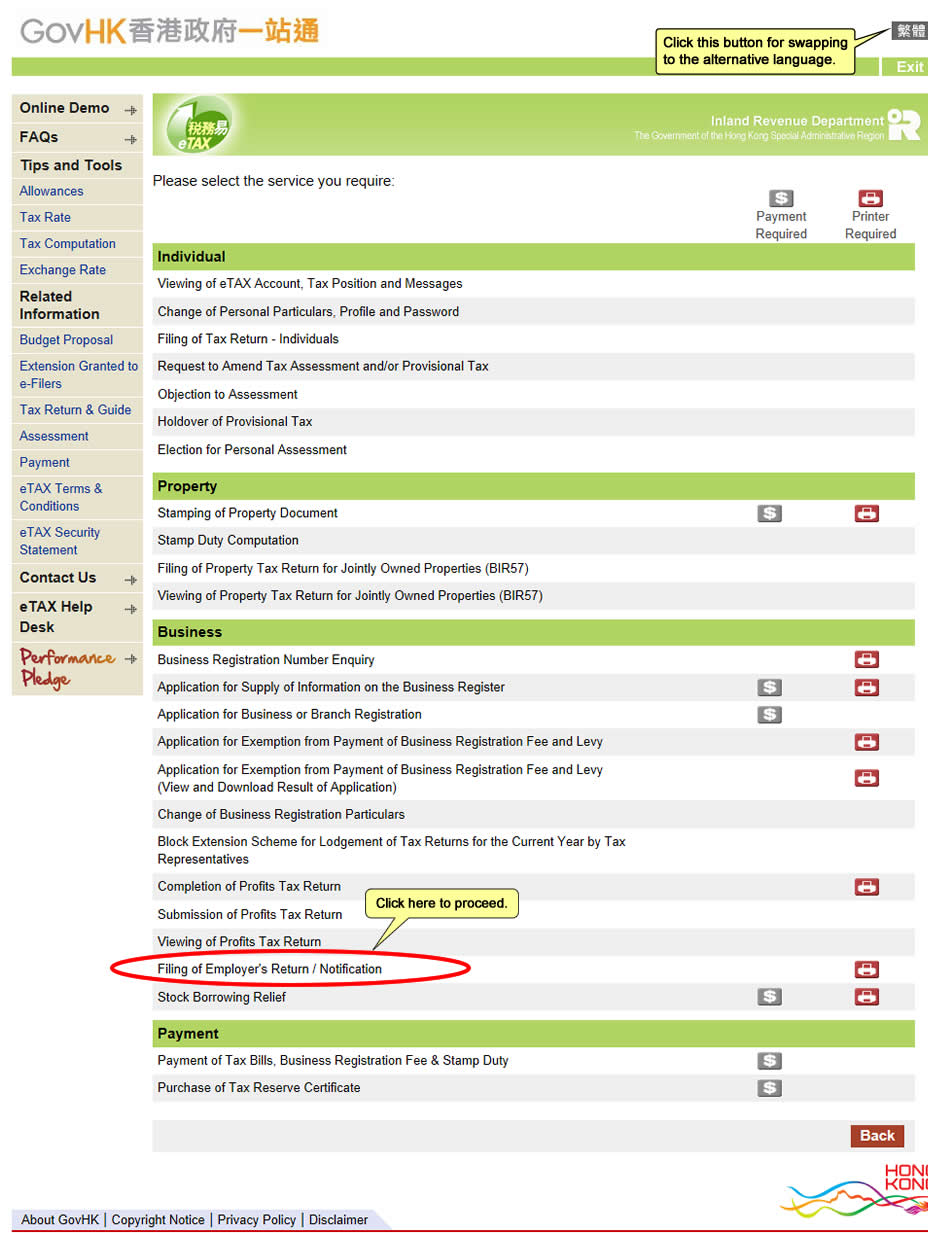This detailed caption provides a thorough description of a screenshot from a government website, presumed to be related to tax services:

---

The screenshot captures a section of a government website, indicated by the "Gov HK" logo at the top left corner. The "Gov" part of the logo is in grey text, whereas "HK" is in a light orange hue. Adjacent to this logo is a version rendered in Asian characters, likely Chinese, given the site's context. The top right corner of the screenshot features more Asian text, with a button allowing users to switch the website's language. This button offers the alternate language option for users preferring a different script.

The website’s layout includes a cream-colored vertical sidebar on the left, housing numerous navigation tabs. These tabs serve various functions and sections of the site, suggesting it is a tax-related website. The top left portion of the sidebar prominently features the word "tax," reinforcing the site's focus. Below this, several additional tabs offer options such as "Online Demo," "Related Information," "Contact Us," and "e-Tax Help Desk," which cater to users seeking assistance or further information on tax returns and related processes. The overall cream background gives the site a clean and professional appearance.

---